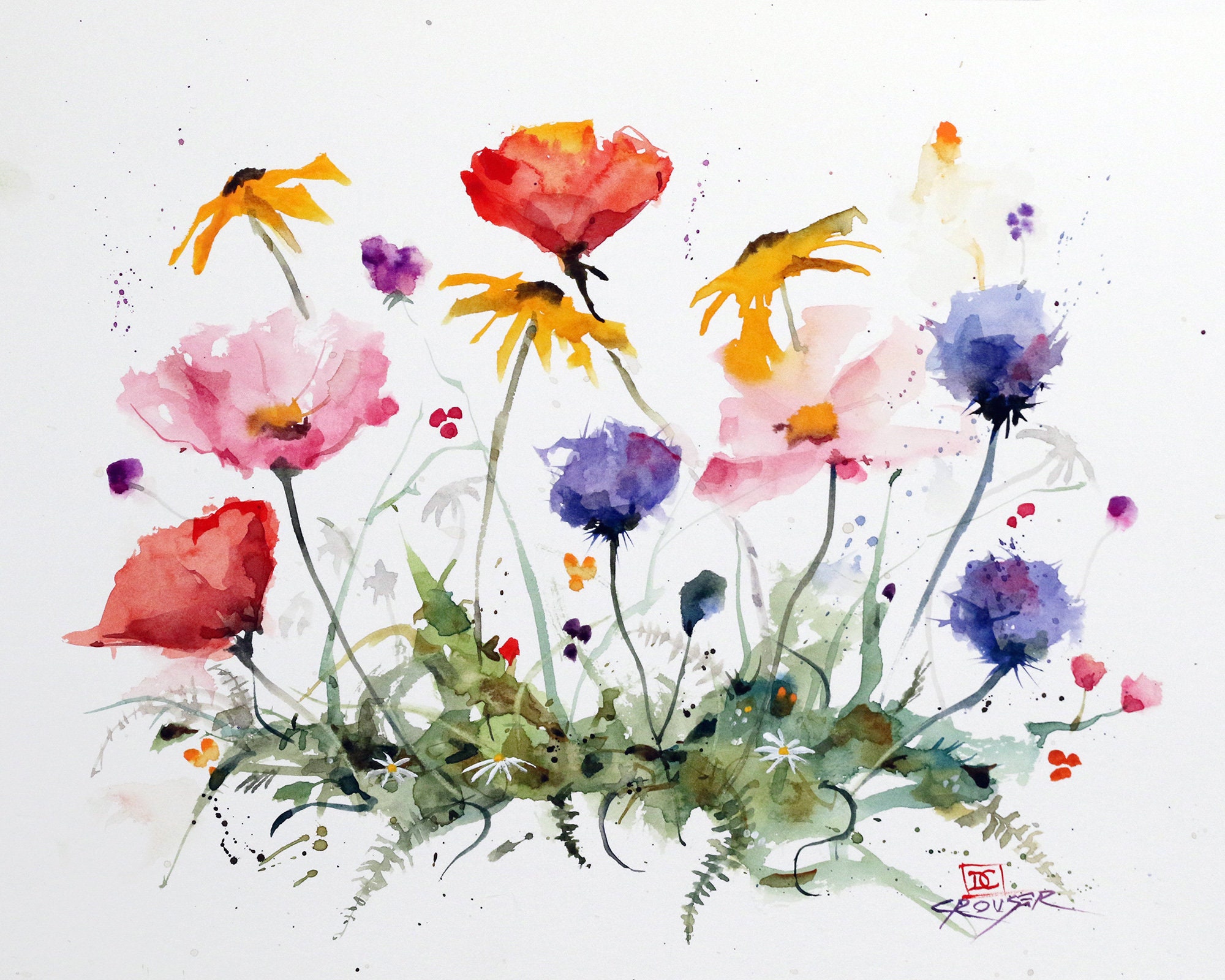This detailed painting showcases a vibrant assortment of wildflowers set against a light gray background. The flowers appear naturally scattered as if growing in a meadow, with various types interspersed throughout. In the bottom right corner, a small red DC logo enclosed in a square can be seen, accompanied by a barely discernible purple autograph. The arrangement includes a dazzling array of colors: cup-shaped red and pink flowers, pink flowers with spread-out petals, blue ball-shaped flowers, and daffodil-like yellow flowers with multiple smaller petals encircling a central brown spot. There's also an array of smaller blooms, such as tiny purple flowers and clusters of yellow, pink, and purple flowers, with green, almost weed-like leaves. Notable individual flowers include a large pink sunflower with an orange center, small white flowers, a singular purple flower, and a red rose. The composition is lush and dynamic, capturing the beauty of wild flora in meticulous detail.